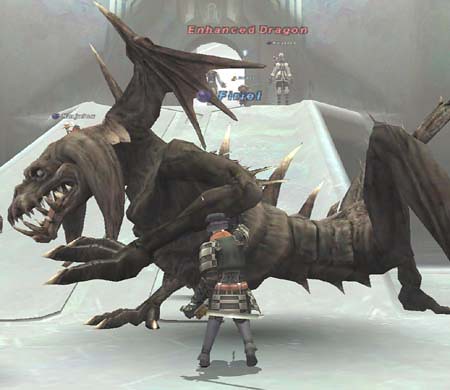In this image, likely taken from a medieval-themed video game, the setting features a dark to light grey gradient sky, transitioning across the scene from the middle out to the sides. The foreground showcases a notably detailed, skeletal dragon, referred to as an "Enhanced Dragon" in red text at the top of the image. This dragon, charcoal grey in color, boasts prominent spikes on its back and belly, and an array of sharp, spiky teeth. It has imposing wings situated on its back, adorned with three spikes at the bottom, and slender legs that each end in three visible toes. A close examination reveals the dragon's head resembling a dog's shape, with long ears and a centipede-like body. 

In front of this intimidating creature stands a warrior, whose back faces the viewer. The warrior wears an elaborately designed armor in shades of grey, detailed with electronic components on the shoulders and a section that appears lighter grey with red accents. This individual also has a blade held behind them and casts a noticeable shadow on the icy ground beneath them.

Further into the background, another figure stands atop what appears to be an icy hill or a mountain. This setting suggests a landscape covered with whitish frost, rising upwards in a gentle ascent. Near the wings of the dragon, there is an inscription in blue, though its complete wording is unclear, possibly reading "flossel" or "floral." The overall image is a captivating blend of dark fantasy elements, enhanced by the game's intricate character designs and chilling atmosphere.